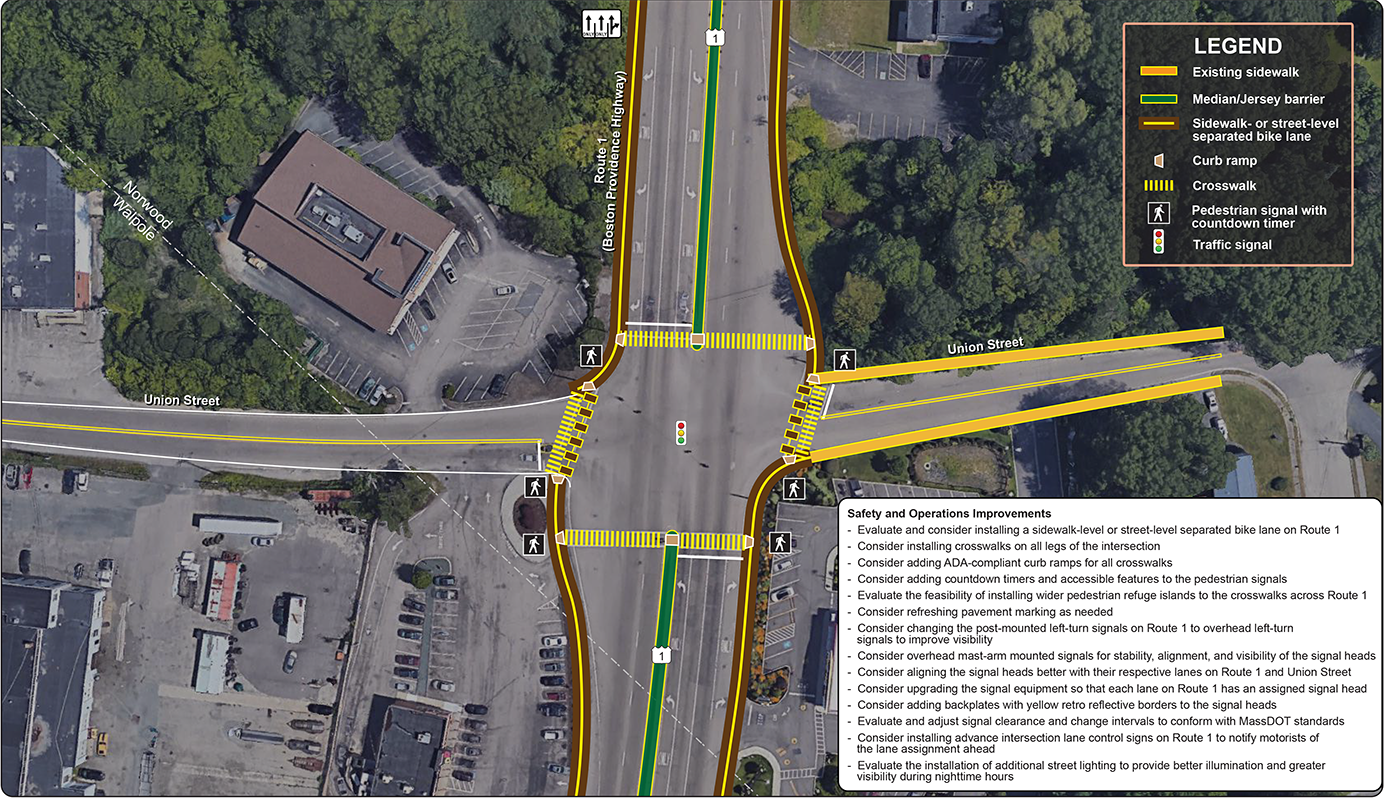The image shows a detailed satellite view of a busy intersection, specifically Union Street and Route 1, Boston-Providence Highway, likely in Massachusetts. The map is enhanced with various symbols and colored lines to denote traffic and safety features. At the center of the intersection, dashed yellow lines indicate crosswalks, while green bars represent medians or Jersey barriers along several road edges. Each side of the intersection has distinct traffic lines and bars, illustrating different safety measures.

In the upper right corner, there is a legend box with a darker, semi-transparent background and an orange outline, which explains the various symbols used on the map. This legend identifies different elements such as existing sidewalks, median Jersey barriers, separated bike lanes, curb ramps, crosswalks, pedestrian signals with countdown timers, and traffic signals.

Additional details highlight safety and operational improvement recommendations for the intersection, including the installation of ADA-compliant curb ramps, countdown timers for pedestrian signals, and refreshed pavement markings. The suggestions aim to enhance the visibility and stability of the traffic signals, improve pedestrian safety, and ensure compliance with MAST DOT standards. The recommendations also include the evaluation of potential benefits from adding advanced intersection lane control signs and improved street lighting for better visibility at night. This detailed map and its annotations indicate that this is part of a MAST DOT project aimed at upgrading the intersection for safety and efficiency.